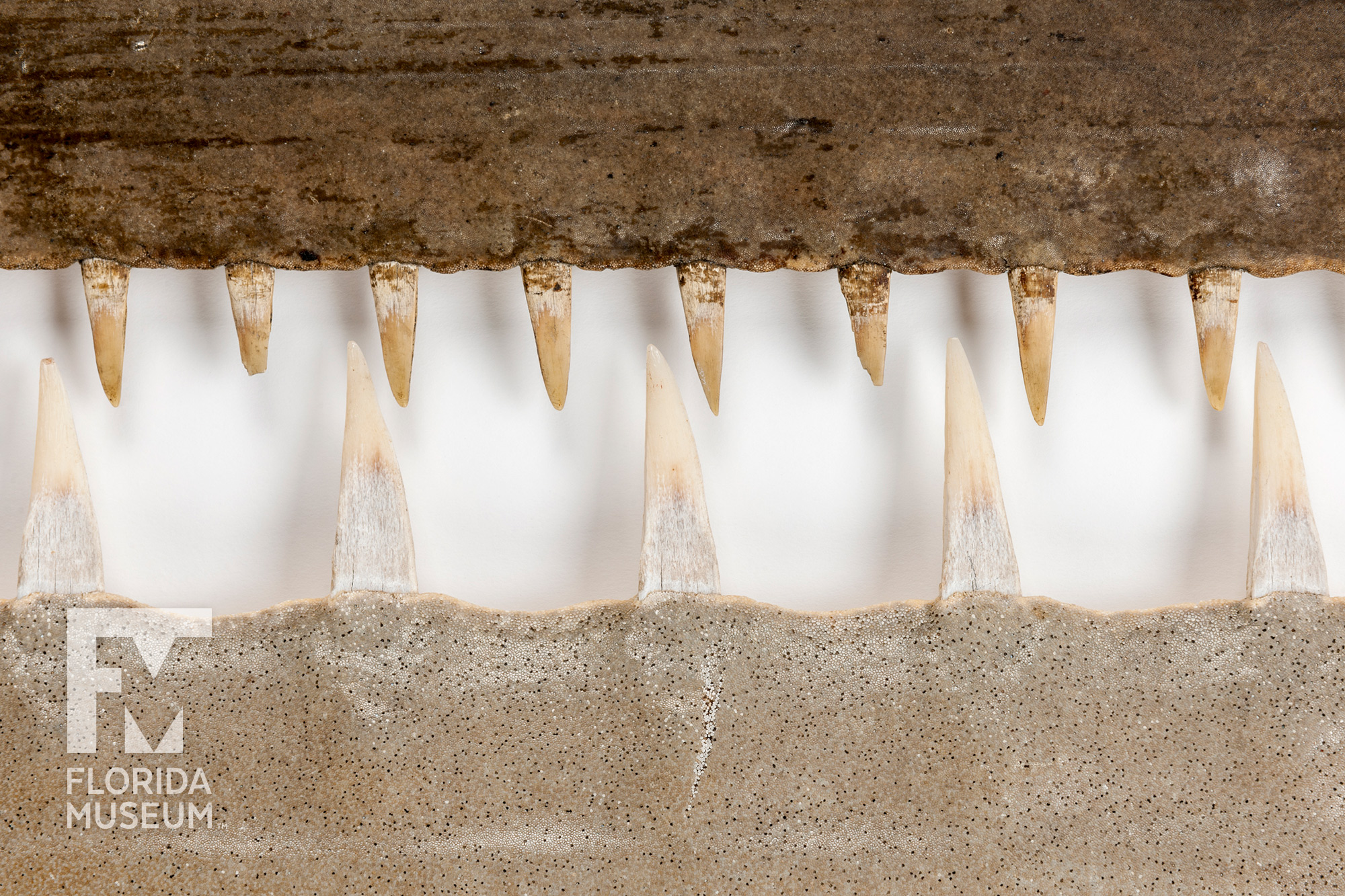This image features a close-up view of what appears to be a fossilized jaw, set against a white background. The fossil consists of two distinct layers of rock, with the top layer being dark and rough-textured, while the bottom layer is gray with white and dark flecks. Protruding from both layers are rows of sharp spikes resembling teeth. The teeth on the bottom layer are tall, sparse, ivory, and white in color, heightened against the light brown of the rock. In contrast, the teeth on the top layer are thicker, shorter, darker, and closely packed, embedded in a darker brown rock with a rougher texture and dirt-like flecks. Some of these upper teeth appear chipped. In the bottom left corner, there is a watermark that reads "Florida Museum" along with its logo.